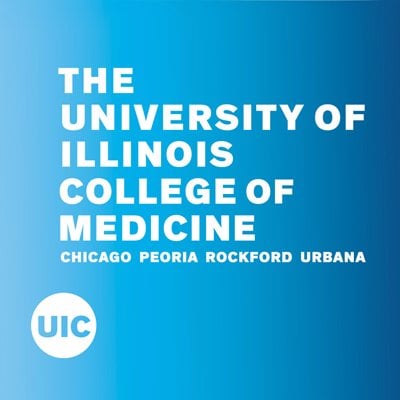Depicted in the image is an intricate design featuring a blue square with the text "White Texas University of Illinois College of Medicine Chicago, Peoria, Rockford, Urbana" inscribed. Adjacent to the blue square, there is a yellow circle positioned over the state of Texas. The left side of the image is bathed in a light blue hue, symbolizing the "bright side," while the right side is enveloped in a darker blue, representing the "dark side." The prominent text within the design emphasizes the presence of the University of Illinois College of Medicine's various campuses: Chicago, Peoria, Rockford, and Urbana. The entire motif is interspersed with these light and dark blue tones to create a visually engaging contrast.